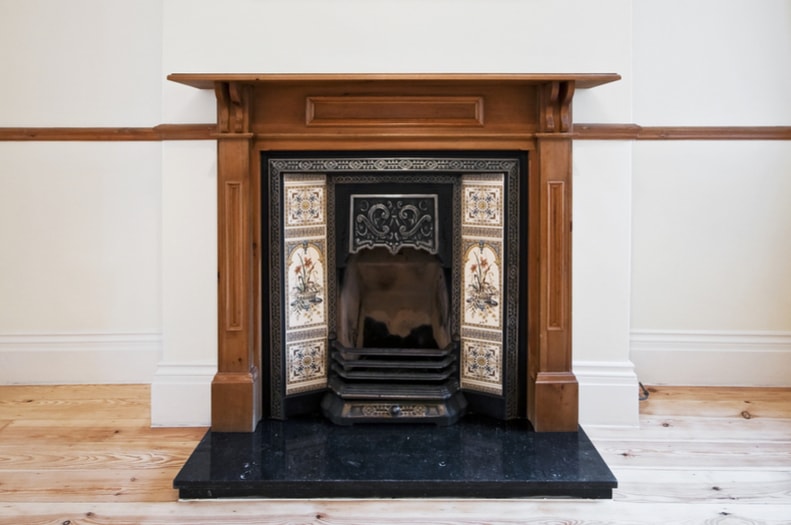This photograph depicts an old-fashioned fireplace situated in an empty, sunlit room. The floors are wooden, and the walls surrounding the fireplace are white, complementing the interior's classic aesthetic. The oak wood mantle, stained a rich brown, features a prominent shelf above the fireplace. The fireplace itself, which is smaller than contemporary designs and resembles a wood stove, is fashioned from metal. It includes a small opening, likely intended for burning coal rather than firewood.

Flanking this central opening are six intricately designed tiles, notable for their ornate floral patterns. These tiles are arranged with four smaller squares on the top and bottom, and two medium-sized squares in the middle. Above the fireplace's opening is a detailed metal design. 

The area directly in front of the fireplace is adorned with black marble, providing a striking contrast to the wooden floor and enhancing the fireplace's vintage charm. The photograph does not include any people or identifiable information about the location or ownership of the house.